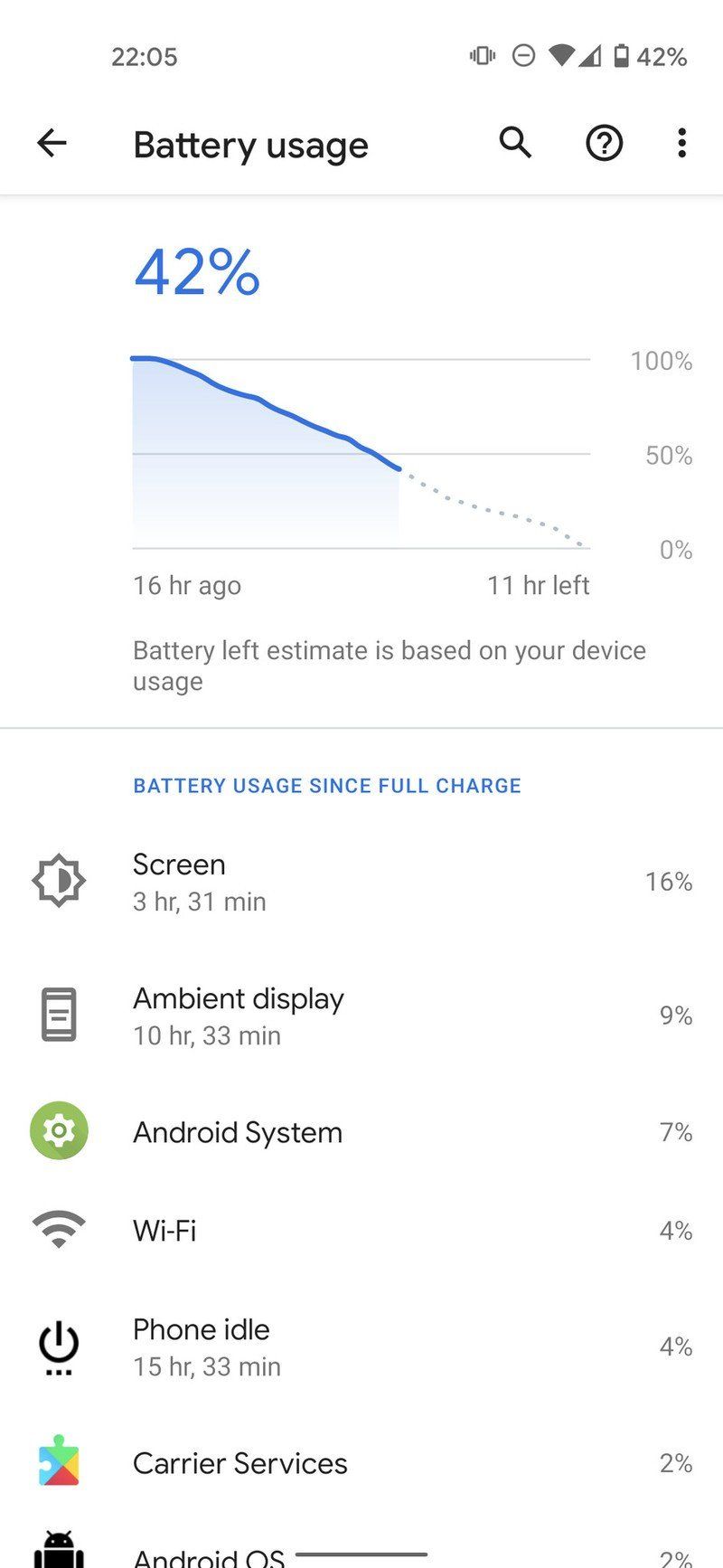This image is a screenshot from a mobile phone, specifically displaying the device's battery usage. The title "Battery usage" is prominently featured at the top left, accompanied by a back arrow to its left and a search icon, a help icon, and a menu represented by three vertical dots to its right, offering additional options or information upon selection.

Below this header, there is a detailed graph illustrating the battery's depletion over time. The current battery level stands at 42%, having declined steadily from a full charge (100%) sixteen hours ago. According to the graph, the device is projected to last another 11 hours before the battery is depleted. A disclaimer beneath the graph notes: "Battery left estimate is based on your device usage."

Further down, the screenshot itemizes various applications and features, listing the percentage of battery each has consumed:
- Screen: 16%
- Ambient display: 9%
- Android system: 7%
- Wi-Fi: 4%
- Phone idle: 4%
- Carrier services: 2%
- Android OS: 2%

This breakdown offers a comprehensive overview of how the battery is being utilized by different components of the device. The screenshot ends with these statistics, completing the detailed battery usage report.